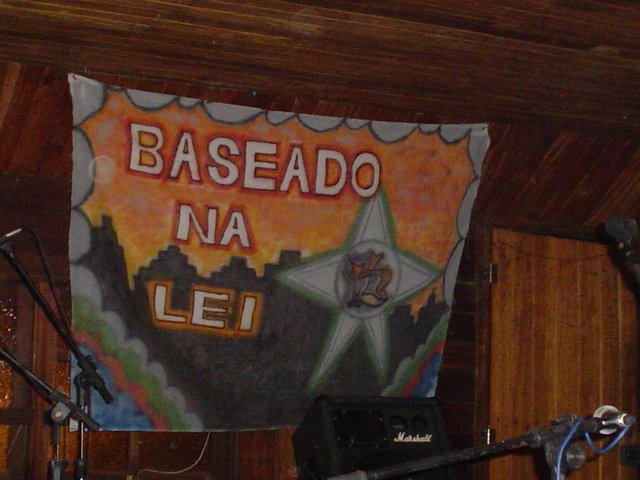This photograph captures a stage set up for a concert, featuring a prominently displayed, hand-drawn banner hanging in the backdrop. The banner, made of fabric and secured at both the roof and possibly the wall, showcases the band's name, Beisadonalei, in white letters outlined with bright red. The lettering emerges from a pattern of colorful clouds in shades of blue, red, green, and lighter green. A star, colored in green and lighter green or gray, rests on one side of the banner. The backdrop includes a vibrantly painted skyline with a gradient of orange, pink, and yellow skies, contrasting sharply with the darkened stage and wooden paneling. The stage setup includes visible details such as wooden doors in the background, a couple of black microphone stands in the foreground, and a black Marshall amp on the floor to the lower right. Overall, the scene is devoid of any people, emphasizing the anticipation of the impending performance.